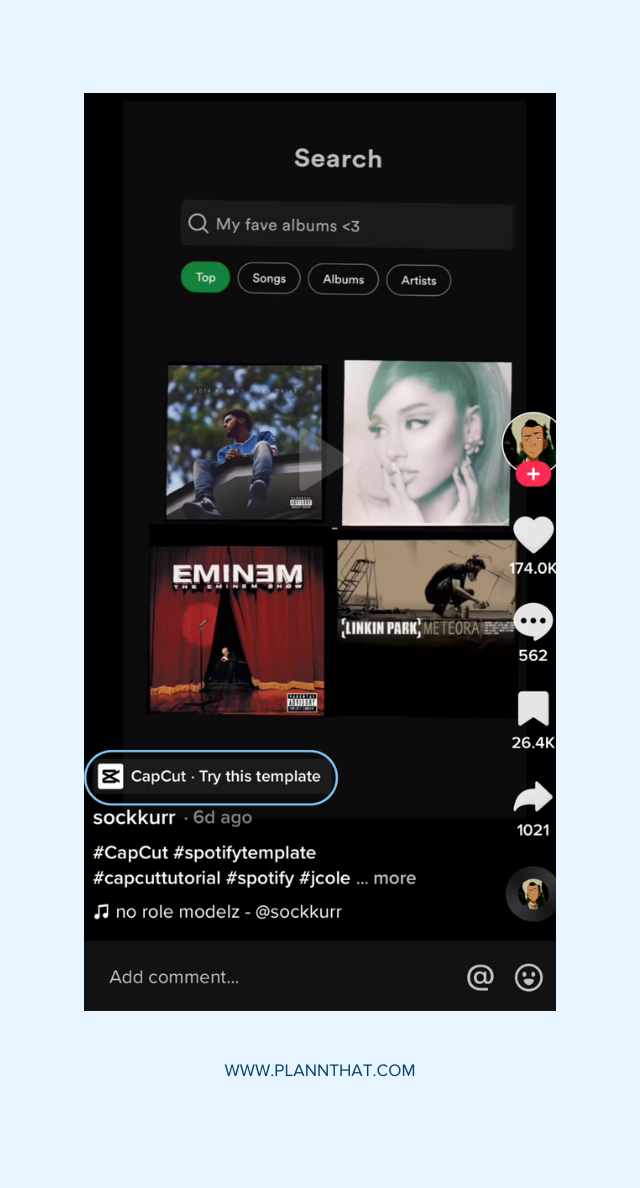This TikTok screen capture showcases a vibrant search interface within Spotify, adorned with various album covers. The background features a light blue hue, setting a calm tone for the image. Dominating the top of the screen is a search bar, labeled "My Favorite Albums" with a heart beside it, highlighted in green. Users can toggle between "Top," "Songs," "Albums," and "Artists," with the current view displaying four prominent albums. 

In the top left corner is J. Cole's album, while next to it on the right is an album by Ariana Grande. Below Ariana's is Linkin Park's album, and to the left of it is an album by Eminem. On the right side of the image, there is a profile picture featuring an anime character, accompanied by various engaging buttons: a like button showing 174,000 likes, a comment button with 562 comments, a bookmark button with 26.4k bookmarks, and a share button with 1,021 shares.

At the bottom of the screen is a prominently circled action button stating "CapCut - Try this template." Additionally, the watermark "www.planthat.com" subtly decorates the bottom of the image. The entire composition offers an inviting snapshot of a user's musical preferences and engagement on social media.